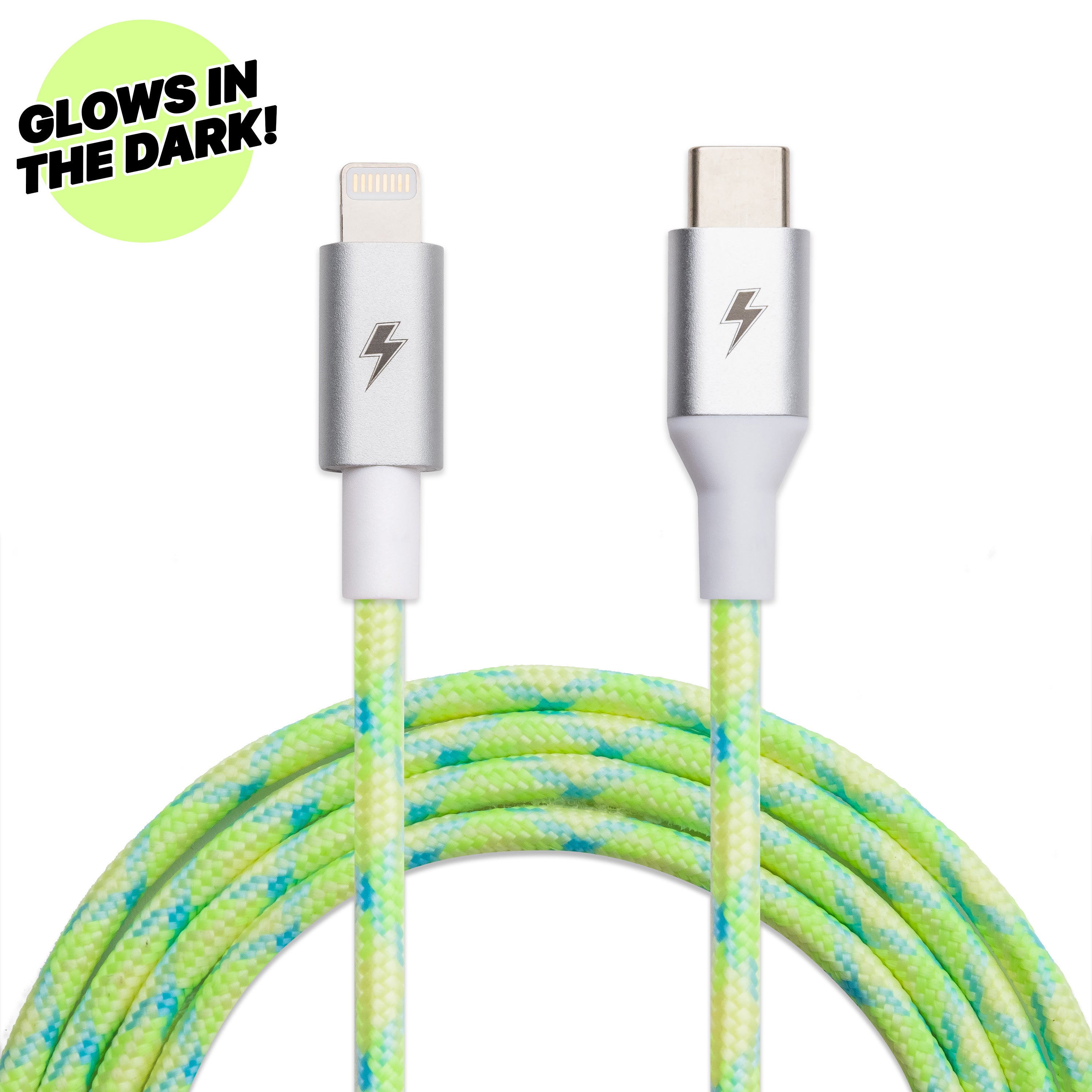In this image, we see two glow-in-the-dark phone chargers prominently displayed against a white background. At the top left corner of the image, there is a label with black text that reads "glows in the dark," set against a lime green circle. The cords of both chargers feature a light green base interwoven with blue dashes, creating a vibrant, eye-catching pattern.

The charger on the left is designed for an iPhone, identified by the distinct lines at its gray end, which also has a black lightning bolt symbol in the middle. Meanwhile, the charger on the right, although identical in color and cord design, has a thicker end with a gray square, indicating its compatibility with a different type of phone. Both chargers possess similar features, yet their ends are specifically tailored for different devices, with each displaying a lightning bolt symbol to signify their function.